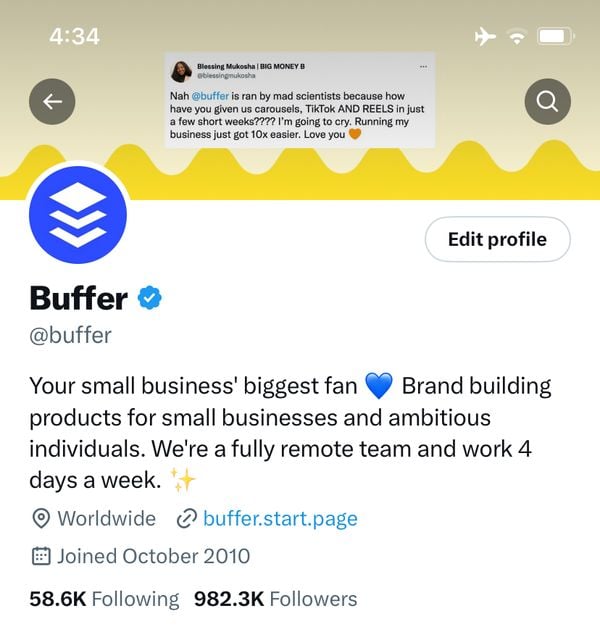The screenshot is from a social media profile interface. At the top, there's a gradient banner transitioning from a grayish-yellow to white, adorned with a wave-like yellow pattern. The upper section contains white text: "434" is displayed prominently on the left, and icons for Airplane mode, Wi-Fi, and Battery are on the right. The left side also features a charcoal-colored circle with a white left-pointing arrow, while the right showcases a similar charcoal circle containing a white magnifying glass icon.

Centered on the banner is the name "Blessing" followed by "Kasha" in capitalized letters and "MUKOSHA" also in upper case. Adjacent to this, "Big Money B" is written in capital letters. The username appears below, followed by a section of text.

Further down, there's a bright blue circular icon depicting three stacked papers. To its right, "Edit Profile" is written with a capital "E." Underneath the blue circle, the username appears again, this time highlighted in black text. Additionally, a teal circle with a white checkmark adjacent to it bears the text "Add Buffer." A descriptive tagline reads, "Your small business is Biggest Fan" accompanied by a blue heart emoji, followed by the statement: "Building Products for Small Businesses and Ambitious Individuals. We're a Fully Remote Team and Work for 4 Days a Week, Worldwide."

At the bottom, there's further information: "Buffer.Start.Page," "Join October 2010," "58.6 Following," and "932.3K Followers."